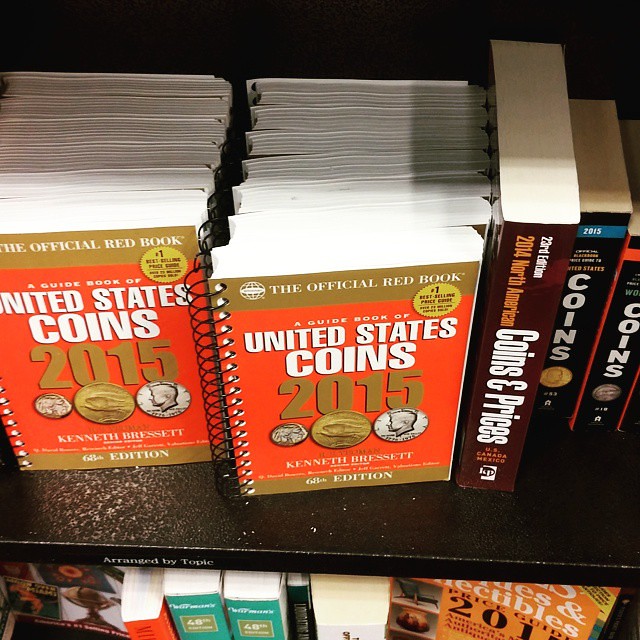The image shows a high-quality, diagonally top-down view of a bookshelf, revealing two rows of books at what appears to be a bookstore. The top row prominently features multiple copies of "The Official Red Book: A Guidebook of United States Coins, 2015," with two books displaying their orange and gold covers to the left and center, while the right side shows the spines of additional copies. The cover of the "Red Book" includes white text highlighting its status as the 68th edition, along with images of a penny, nickel, and dime. To the right of these, several other books on coin collecting are lined up, including a taller book titled "Coins and Prices." Below this row, another shelf is visible with more books, although their details are mostly out of view. Notably, a sticker on the shelf mentions that the books are "Arranged by Topic."